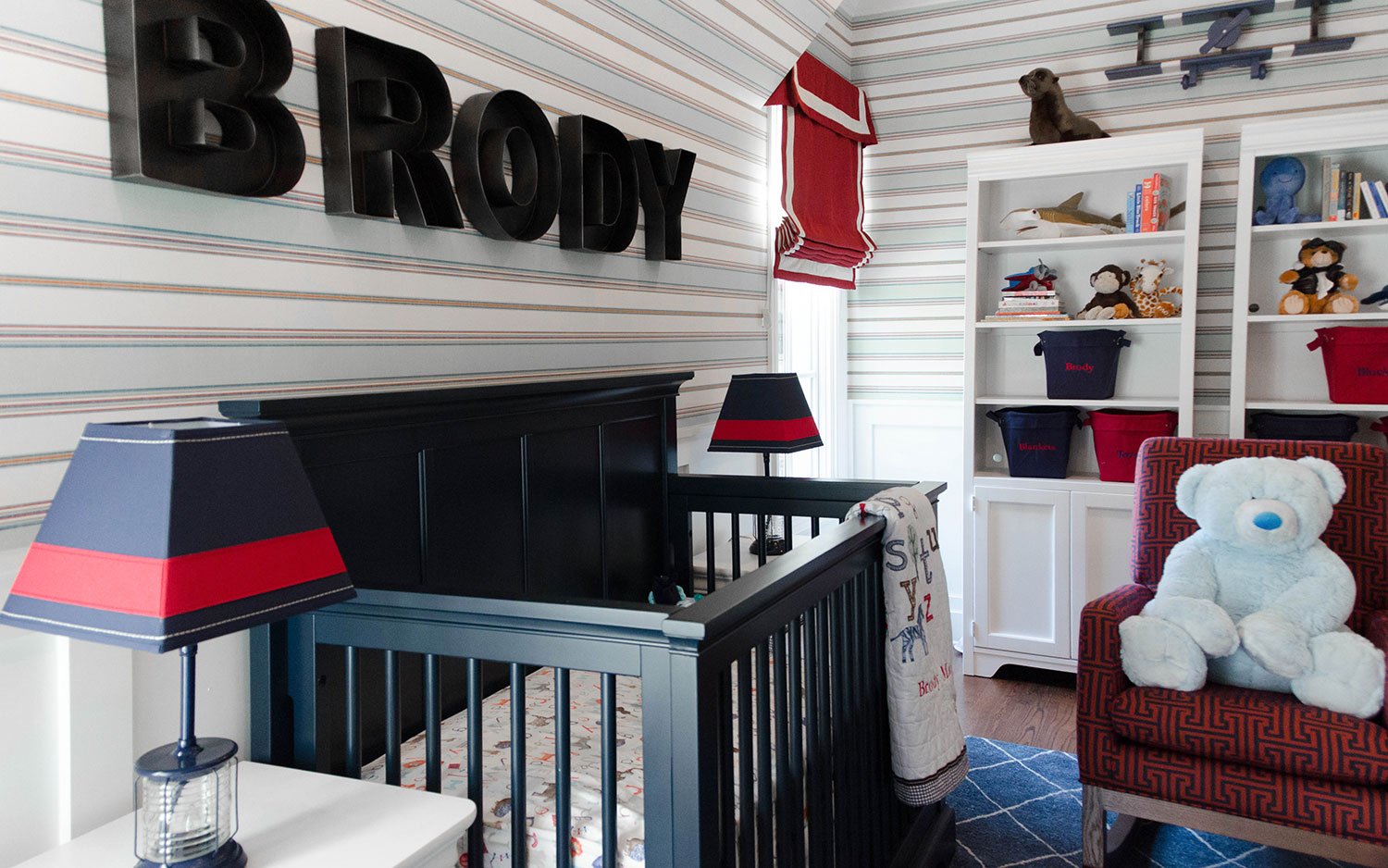The indoor daytime photo captures a meticulously decorated baby's room, showcasing a combination of light blue, white, dark blue, and accents of brown, red, and gold. Central to the composition is a black crib with a white mattress, adorned with a blanket featuring letters and animals hanging over the edge. The wall above the crib proudly displays the name "Brody" in large, black block letters. Flanking the crib are two white nightstands each topped with a glass-based lamp featuring a blue shade with a red stripe.

To the right of the crib, there is a red chair designed with a Byzantine-style pattern, holding a large light blue stuffed bear. The back wall of the room displays a striped wallpaper in light blue, white, and gold with thin red lines. The room includes shelves filled with children's books, toys, and stuffed animals, including a seal and a shark, adding to the playful and warm atmosphere.

The setting suggests it is a carefully put-together space for a newborn, with ample daylight enhancing the cozy, welcoming ambiance of Brody's nursery.